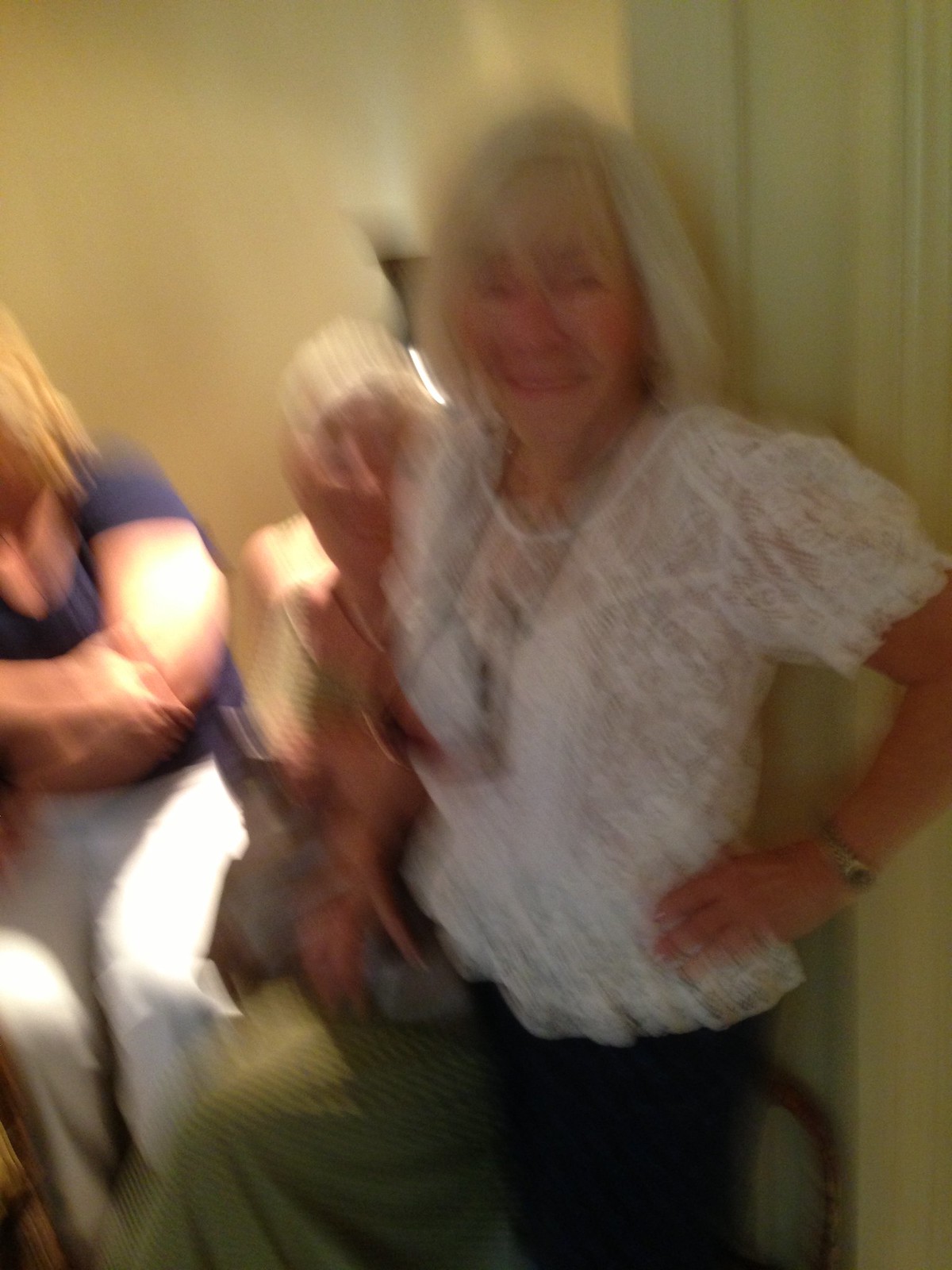This is a blurry, color photograph depicting three individuals inside a room with light gray curtains and a yellowish background. In the forefront, an older woman with short, shoulder-length white or blonde hair, smiles directly at the camera. She wears a white, lace-like, short-sleeved top and dark pants, and has her hand resting on her left hip, adorned with a gold-style watch on her left wrist. To her right, partially visible, is an elderly man with gray hair, only partially seen behind her. To her left, another woman is present with her torso visible but face obscured. She has shoulder-length blonde hair peeking out from under a short-sleeved blue shirt and light-colored pants, with her arms crossed.